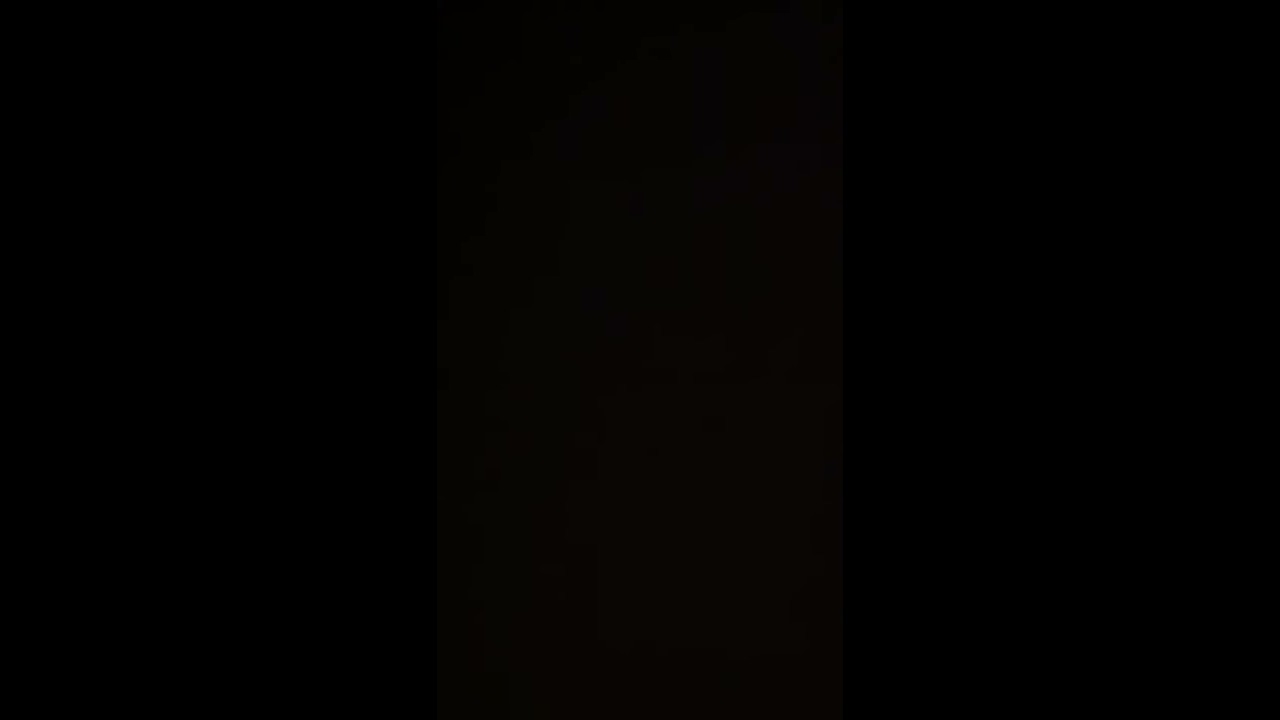In this image, we observe a completely black rectangle. Dominated by a solid black color, the image does not contain any objects, text, designs, or people. The entire composition is just a uniform expanse of black, potentially hinting at a technical issue or an intentional artistic statement. The only subtle variation might be a slightly lighter shade of black centrally located, though this is extremely subtle. The rectangular shape of the image, which is longer vertically, gives a portrait-like appearance. Despite the uniformity of the black, some minor compression artifacts may be present, adding slight texture amid the otherwise homogeneous color. The overall effect is one of a profound, uninterrupted darkness, as if rendered in a setting devoid of any illumination.